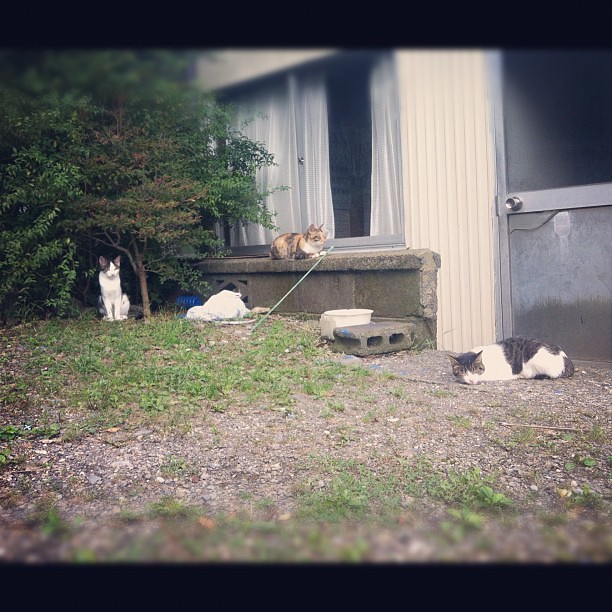The image is a vibrant outdoor scene showcasing the side of a white house adorned with large windows featuring light gray, metallic-looking curtains—one set fully covered and the other spread open. A door with a black upper panel, silver lower portion, and a silver knob is situated prominently. Beside the door, a grayish-brown tabby cat is curled up, sleeping soundly on the ground. To its left, a cinder block and a white bucket are positioned nearby. Adjacent to these, a white dog faces away, next to a blue plastic bucket. Further left, a tall, black and white cat sits upright under some trees and bushes. In front of a concrete ledge under the windows, a calico cat with shades of brown, light brown, and white lounges comfortably. Nearby on the ground, a white cat with black spots sprawls out with its head turned away. There's another white cat with black markings around its ears sitting close to the ledge. The ground is a mix of brown dirt, sparse grass, and scattered greenery, featuring some bright green and brownish-red leaves. Additionally, some cinder blocks and bags, possibly containing construction or gardening materials, lay scattered across the dirt.